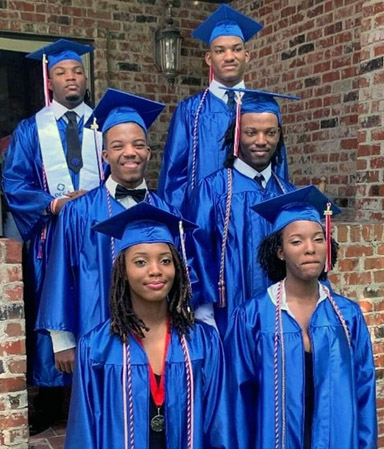This is a detailed photograph featuring six young African students, who have just graduated from high school or college, all beaming with happiness. They are dressed in royal blue graduation caps and gowns, each adorned with red and white tassels. One of the students in the back left is notably wearing a white sash, signifying an honors award. They are arranged on brick steps in front of a brick building, perhaps a house, with a window and an exterior lamp visible in the background. The two females stand in the foreground on the lowest steps, while the four males are positioned behind them, two on the middle steps and two higher up. The group is clearly enjoying the daytime celebration, their bright smiles captured against the rustic brick backdrop.